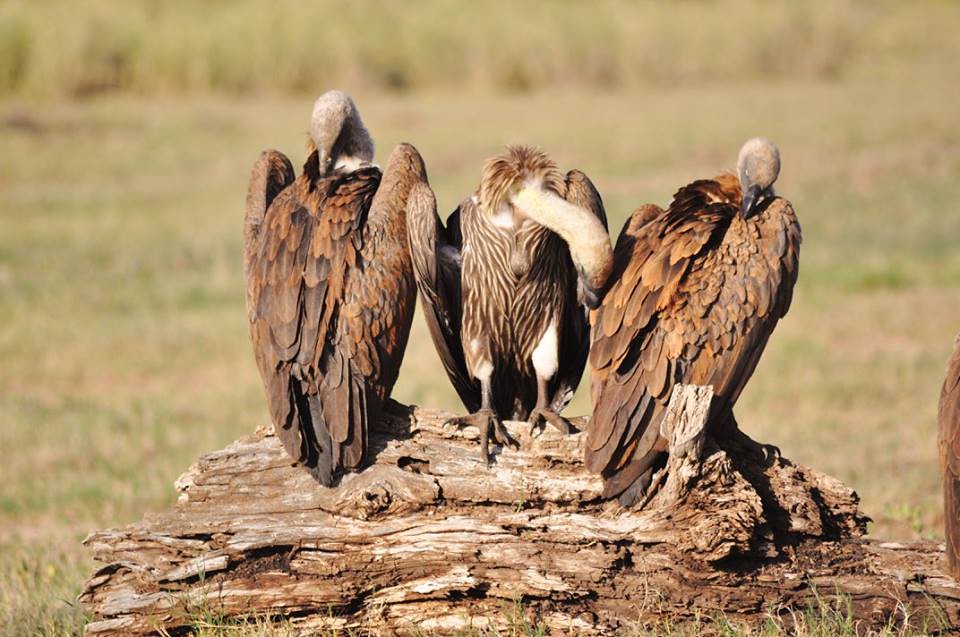In this detailed outdoor color photograph, three large vultures are perched on a decaying, weathered log. The vultures, identifiable by their mostly featherless necks and heads, have brown feathers interspersed with small, fluffy feathering patterns, particularly on their legs. Their coloration closely matches the log they are standing on, providing a natural camouflage. The two vultures flanking the sides have their backs toward the viewer and are preening themselves, with their necks twisted backward. The vulture in the middle, distinctly facing the viewer, reveals a striped chest pattern and prominently visible white, fluffy feathering on its legs along with sharp talons gripping the log. The background is soft-focused, showcasing a blend of brownish-green grass, suggestive of a drying savannah, and denser, green vegetation in the distant blur, adding depth to the natural habitat depicted.